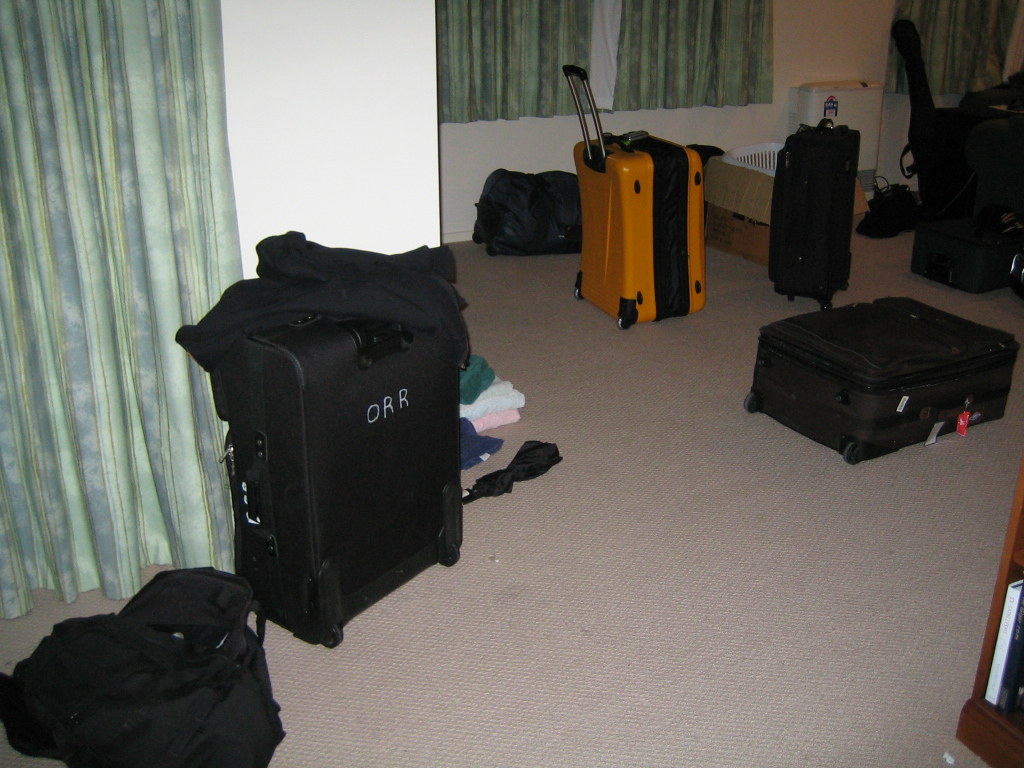The image depicts a cluttered hotel room with suitcases strewn across a beige carpeted floor. The room features white walls and multi-toned green and blue striped curtains that hang over windows, with the curtains on the left extending all the way to the floor and those in the back center stopping about two feet above the floor. Several pieces of luggage are scattered around, most of which are black. Notably, one black suitcase stands with the initials "O-R-R" in white lettering. There is also a hard shell orange briefcase with a black center band, as well as a distinctive yellow and black suitcase standing prominently almost in the middle of the picture. Some luggage bags are laid flat while others stand upright. Additional items include a cardboard box, a guitar case in the background, and various articles of clothing draped over the luggage and lying on the floor, as well as a black umbrella.